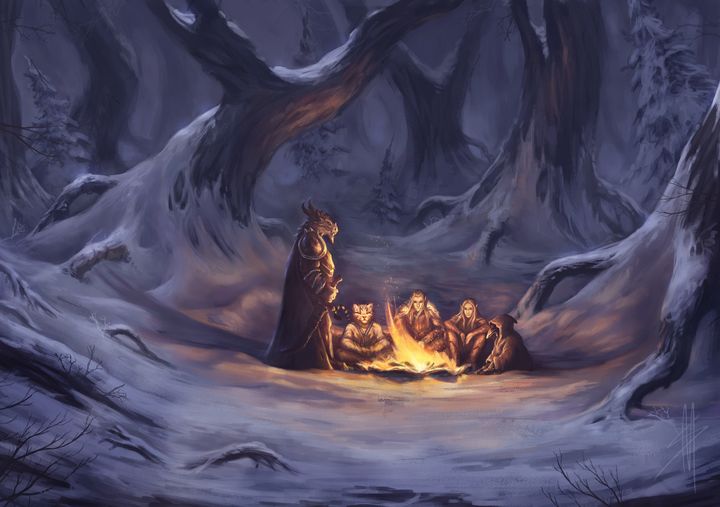The image is a rectangular, artist's graphic sketch with a dark, fantasy-like ambiance, featuring a group of fantastical creatures gathered around an upright yellow campfire. The scene is set in a snow-covered, dense forest with tall trees cloaked in shadows and an overall purple tint dominating the view. Central to the composition, four figures are seated around the fire, each wrapped in cloak-like garments. Noticeably distinct, one figure boasts a human body with a cat's head, another has a human face with pointy ears and long hair, the third appears human-like with pointy ears, and the fourth is partially hidden, displaying a raven's beak peeking out from a cloak. To the left stands a figure in a warrior's cloak, holding a sword, characterized by a devilish face with horns or possibly a dragon-like visage. The figures are bathed in the fire's flickering light, creating a mysterious and eerie atmosphere, with no text or wording present in the image, enhancing the viewer's focus on the detailed, otherworldly scene.